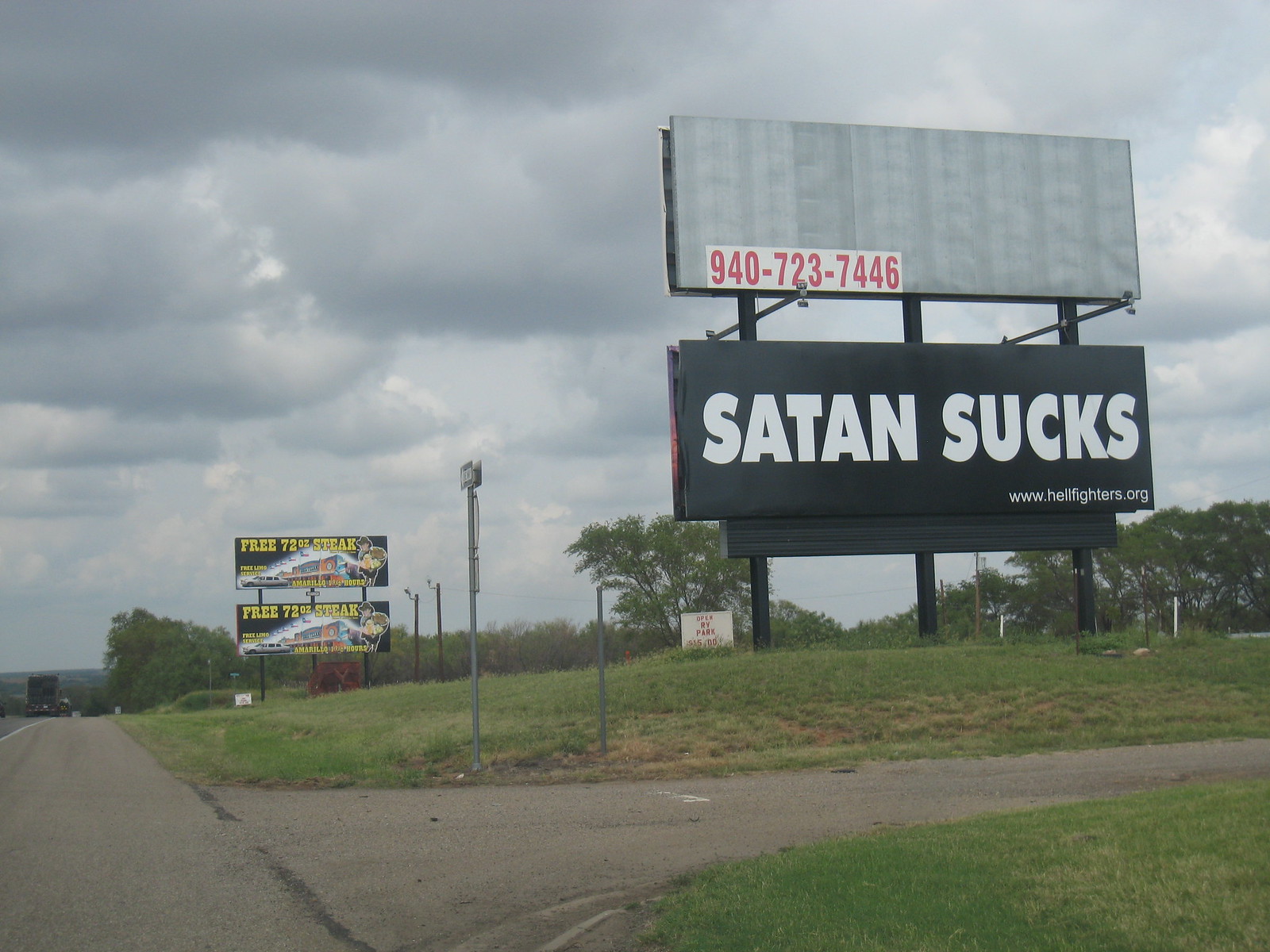A winding road curves to the right, forming an L shape, with lush green grass lining both sides. Alongside the road, a pair of billboards stands out amid scattered trees. The sky above is a medium shade of blue, dotted with plentiful white clouds.

The top billboard is painted light gray, with a conspicuous red phone number "940-723-7466" displayed at the bottom. Below it, a black billboard reads "Satan Sucks" in bold white letters, along with the website "www.hellfighters.org."

Adjacent to these, another set of billboards mirrors the first pair. The top sign advertises a "Free 72 oz Steak." The overall scene is rich with outdoor elements and a touch of promotional flair, where nature and advertising coexist.